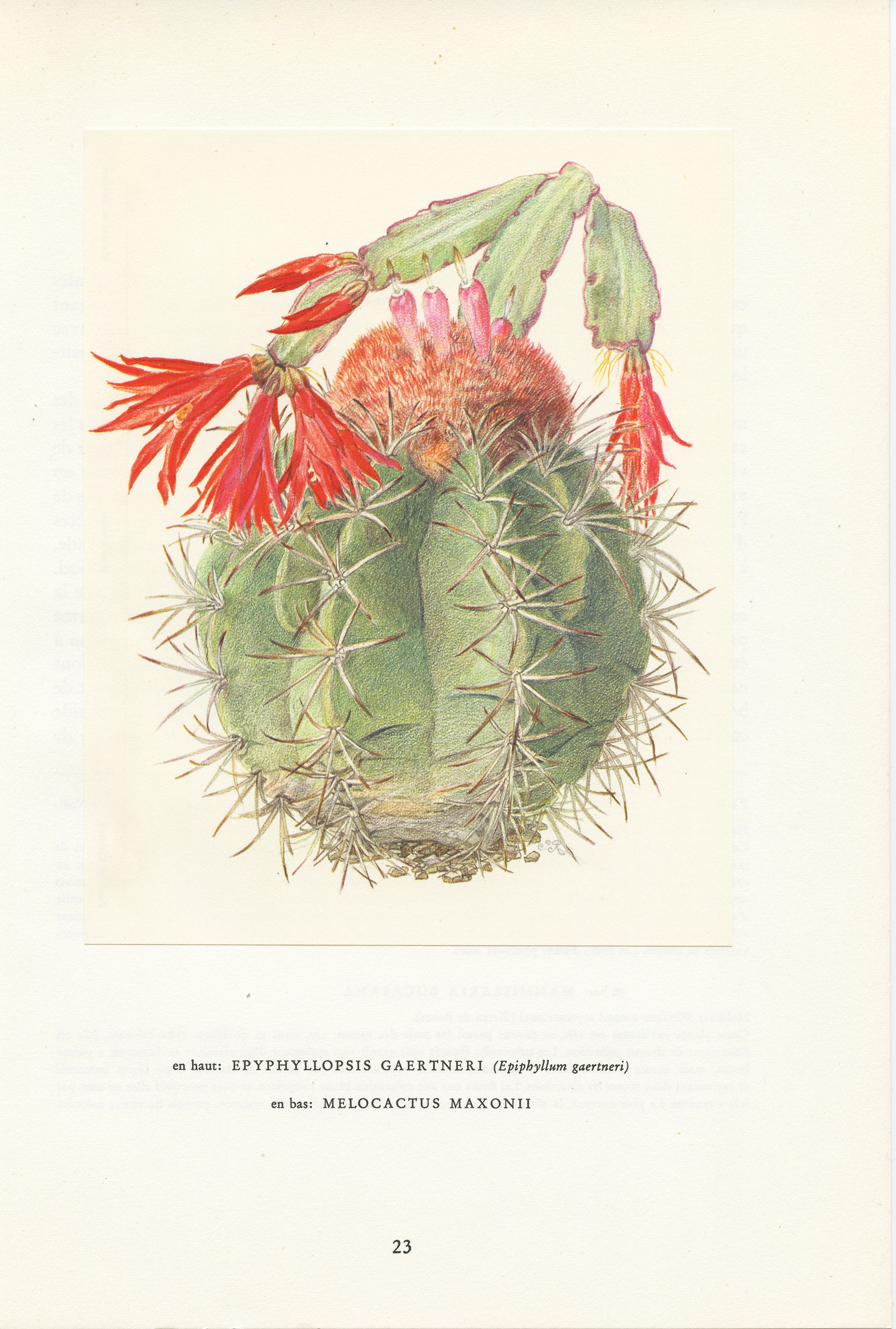The image depicts a detailed botanical drawing of a cactus fruit, specifically identified as Epiphyllum gardneri and Melocactus maxonii (noted in the accompanying text), against a white background. The plant has a slightly circular form with multiple green stems extending outward, each adorned with small prickly spines. At the top of the cactus fruit, there is a furry or bristly red-topped surface from which small pink flowers sprout. Red flowers are seen blooming from the tips of three branching segments, with one branch partially obscured behind the main cactus fruit. The composition also includes some yellow and brown elements at the base, indicating roots or parts of the plant's lower structure. The bottom of the image contains a typed description, including the line number 23, which likely references the page from which this botanical illustration is sourced.